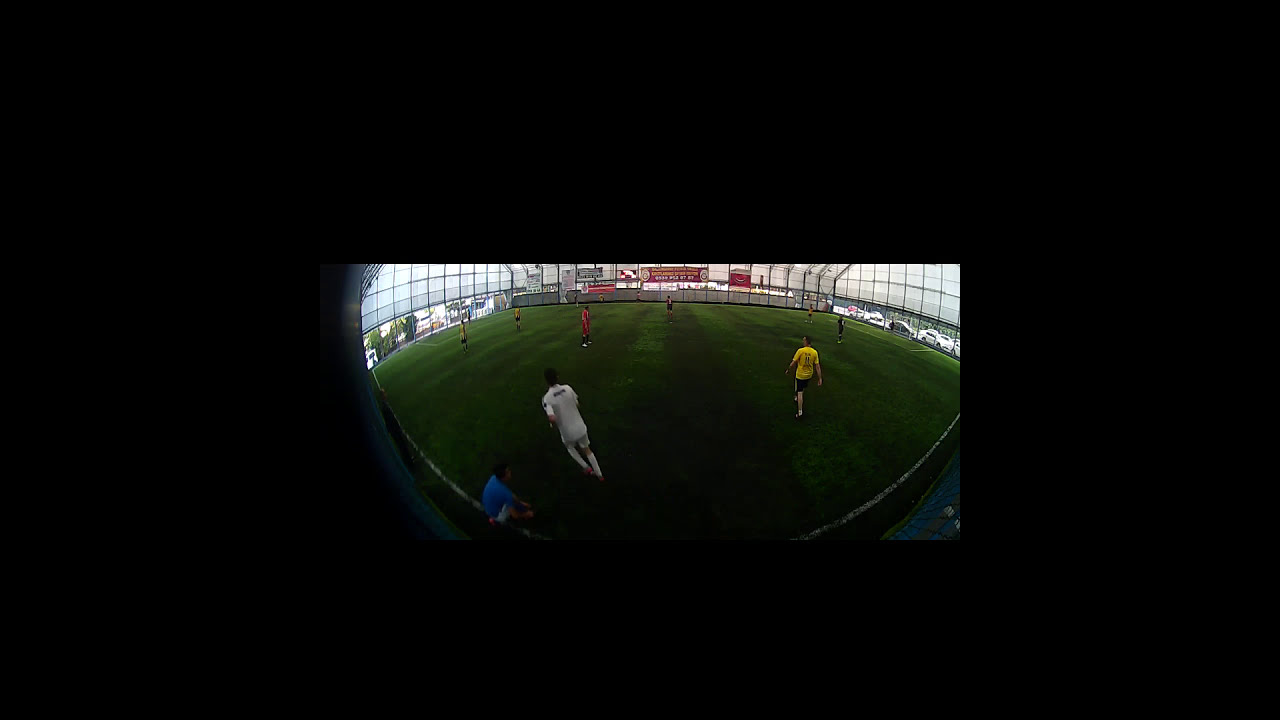The image depicts an indoor soccer match or practice session, characterized by its vibrant and dynamic setting. The field is lush green, meticulously mowed in a recognizable pattern, and enclosed within a substantial dome-like pavilion made of plastic or glass, featuring square-patterned windows on either side. This enclosure allows a glimpse of cars parked outside on the far right. The photo itself has a fisheye lens quality, giving it a slightly distorted, rounded appearance.

In the scene, multiple players are visible, wearing diverse jerseys: red, yellow, and white, suggesting mixed teams or a practice session. In the foreground, a man in a blue shirt is seated on the grass beside a standing man dressed in all white. Nearby, a player in a yellow shirt with black shorts is captured in motion. Further into the field, additional players are seen, one notably in red. Surrounding the playing area are several advertisements mounted along a fence. The overall setting suggests a vibrant, active sporting environment within a well-maintained facility.